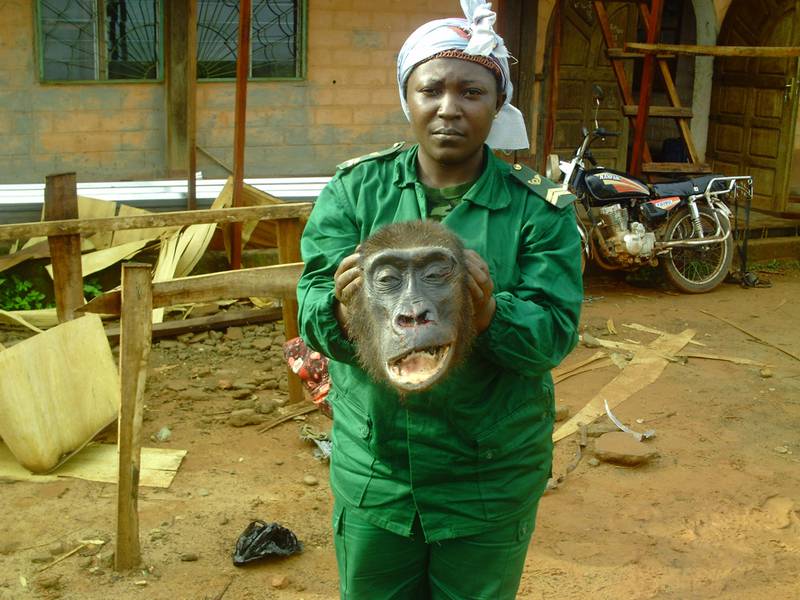In this detailed image, a black woman is seen wearing an all-green military uniform, complete with official-looking military bars on the shoulders. She has a light blue cloth tied around her head, with the frayed ends of the material visible. The woman is holding up, between her hands, the severed head of what appears to be a gorilla, gruesomely displaying it for the camera. Behind her to the left, there are large, dried leaves and scattered boards, suggesting a scene of disarray. To the right side of the background, a black motorcycle is visible, adorned with rust-colored labels. Further back, there is a brick building with a doorway on the upper right side and a window on the left side. The ground around her is littered with strewn bits of wood, veneer, and debris, adding to the chaotic atmosphere.